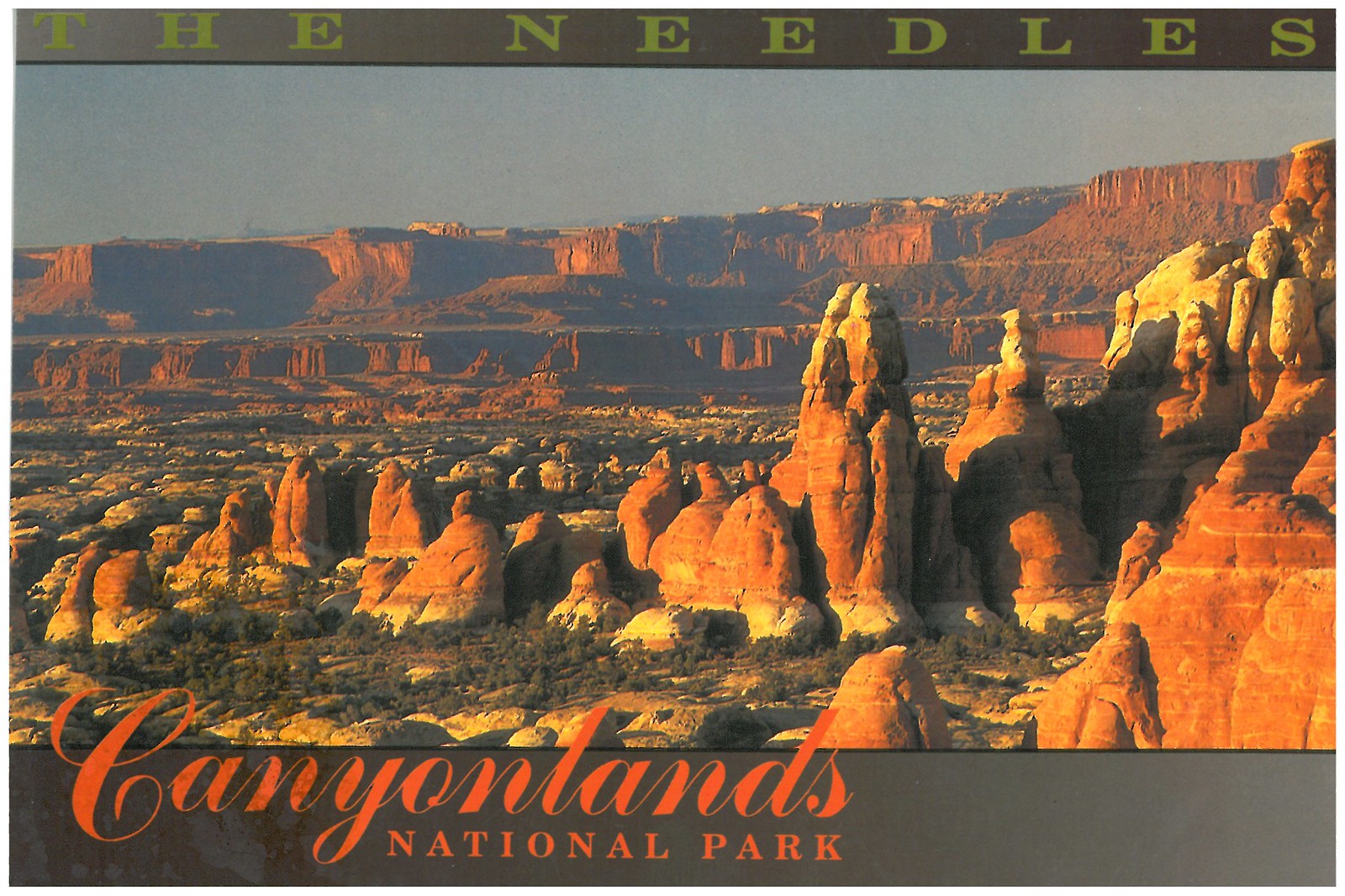This image depicts a striking scene at Canyonlands National Park. Featured prominently is an array of elaborate, oblong rock formations rising from the valley floor under the warm orange hues of late-day sunshine. The backdrop reveals a series of cliffs, layered one behind another, under a blue-gray sky. Vegetation is scattered at the base of some of the towering rock structures, adding a touch of green to the predominantly reddish-orange landscape. The image is formatted like a postcard or a calendar page, with a thin taupe band at the top and a thicker one at the bottom. The top band displays the text "The Needles" in light green, while the bottom band, overlapping parts of the rock formations, features "Canyonlands National Park" in orange script that partially extends above the band. The overall scene captures the grandeur and rugged beauty of this iconic national park, devoid of any human presence or man-made structures.